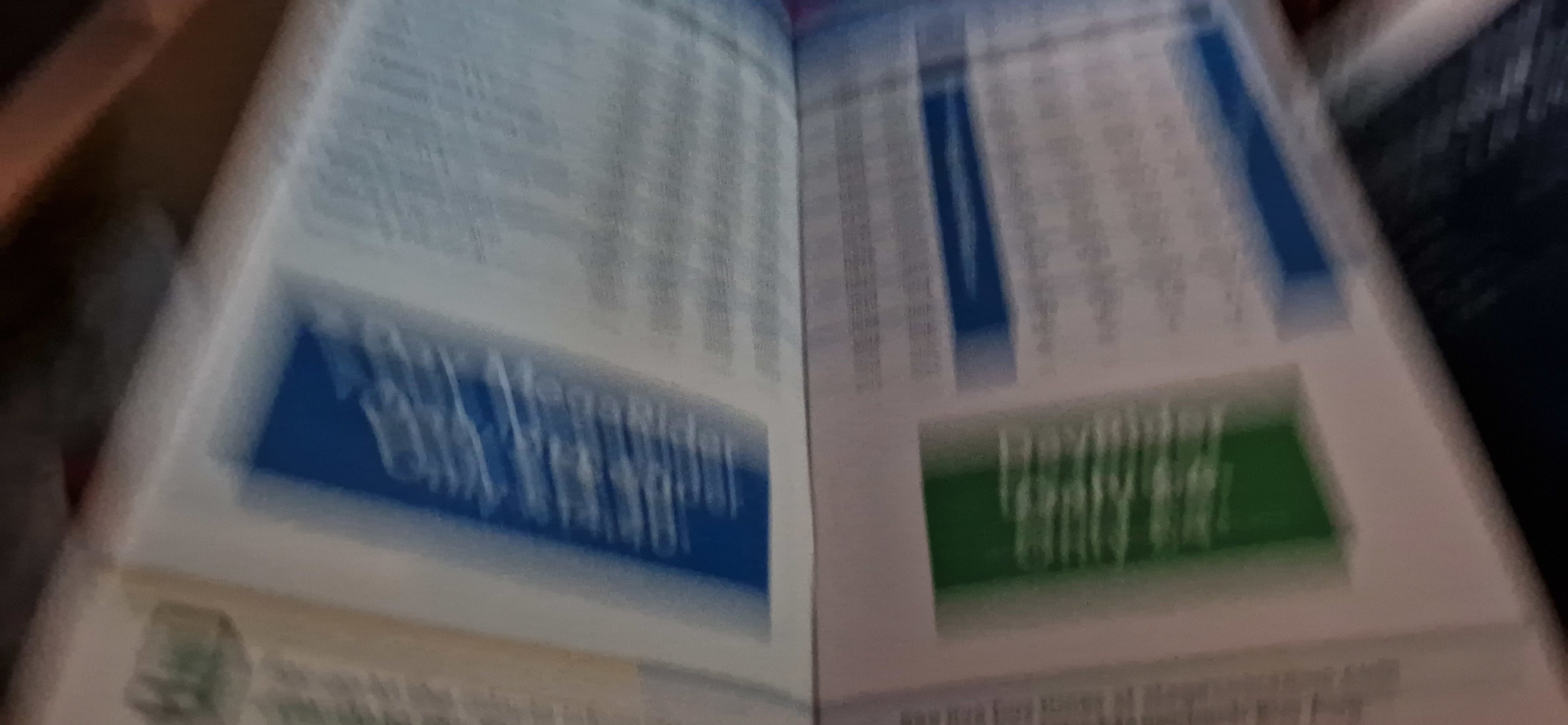The image is a highly blurry photograph of an open booklet or instructional type booklet, making most of the content indistinguishable. On the left page, there is a large blue rectangle with white writing that appears to contain a title or heading, possibly reading "Mega Rider." The right page features a similar layout with a green rectangle at the bottom, likely containing text, possibly including the term "Day Rider." Both pages seem to have some form of writing or tables of data above the rectangles, potentially multiple-choice questions, but the blur obscures any clear detail. The bottom of the image shows an extended, partially cut-off, and indistinct portion of the booklet. The background flanking the booklet is slightly visible, showing some color variations.